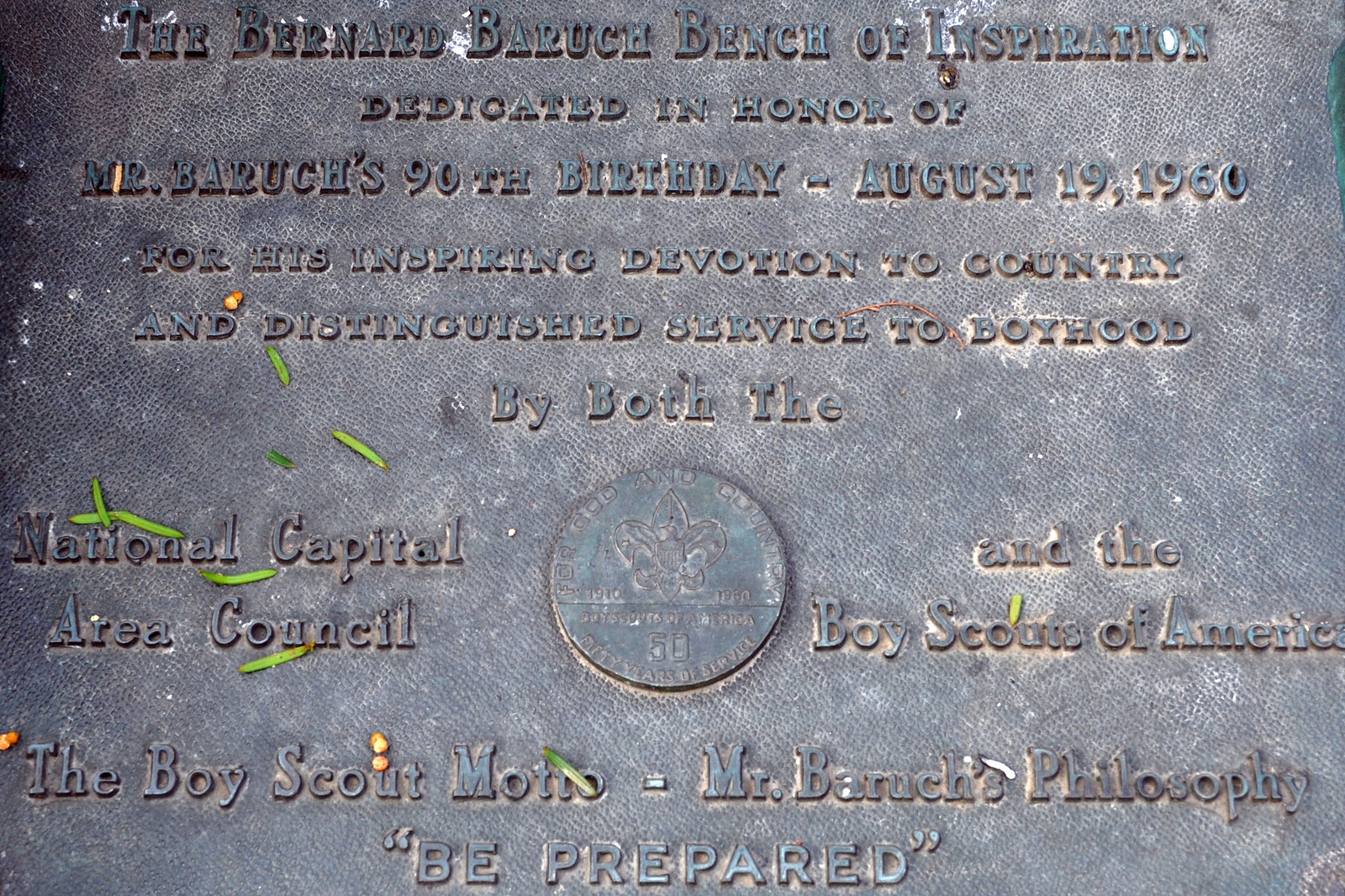This is an overhead color photograph of a bronze plaque with raised, etched text. At the top, the plaque reads, "The Bernard Baruch Bench of Inspiration," in capital letters. The plaque is dedicated in honor of Bernard Baruch's 90th birthday on August 19, 1960, and it celebrates his inspiring devotion to his country and distinguished service to boyhood. Centrally located on the plaque is a circle containing a Boy Scout logo with a Fleur de Lis and the number 50. To the left of the logo, the text reads "National Capital Area Council," and to the right, "Boy Scouts of America." At the bottom, the plaque connects the Boy Scouts' motto with Mr. Baruch's philosophy: "Be Prepared." The plaque's bronze surface shows signs of discoloration, adding to its aged appearance.